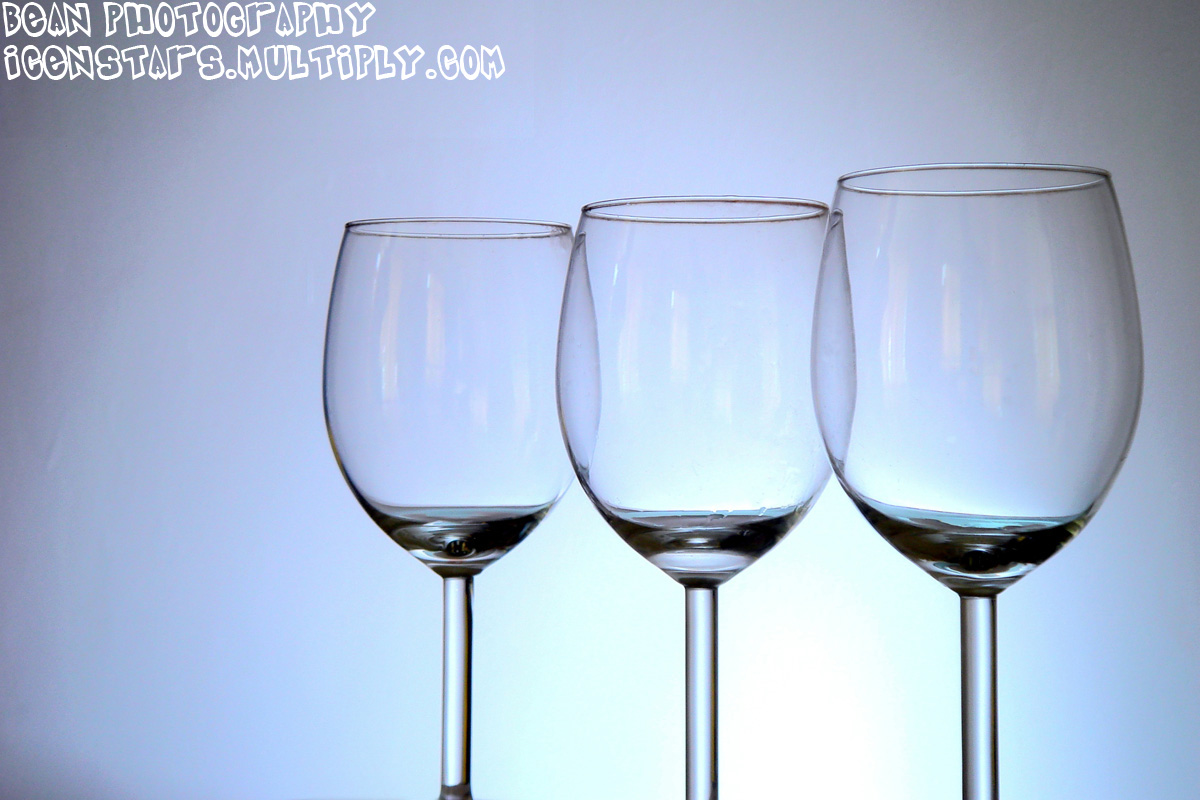The image captures three transparent glass wine glasses, each with approximately 10 milliliters of a clear liquid, aligned from left to right centrally in the photograph. The glasses, appearing uniform in size and shape, are positioned obliquely, allowing for a slight reflection of light off their surfaces. The backdrop is predominantly slate blue with a noticeable glow emerging from below the middle section, creating a gradient effect where the upper corners and bottom areas appear darker. Above the glasses, in a white bubble font, the text "Bean Photography" is prominently displayed, followed by the website "ekanstars.multiply.com" in smaller, white letters. The overall lighting and composition lend a serene ambiance to the photo, emphasizing the elegance and simplicity of the glassware against the subtly illuminated background.